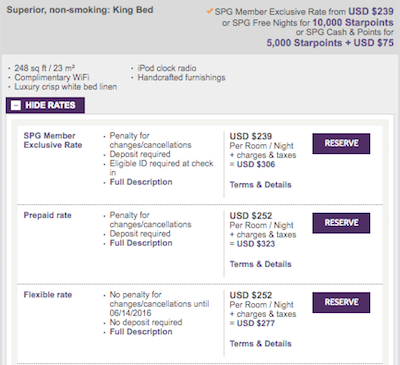The image depicts a hotel room booking aggregator, likely from the Starwood hotel chain, given the references to Starpoints, the loyalty program commonly associated with Starwood. The website has a predominantly gray color scheme, complemented by darker, almost purple boxes that highlight key information, and purple font used for accentuating specific details.

The user has conducted a search for a superior non-smoking room with a king bed. The results page indicates both the number of Starpoints required for booking and the additional monetary cost. Beneath the top-line menu that provides this summary, a detailed list of room features is displayed. The room offers 248 square feet of space, complimentary Wi-Fi, crisp white bed linen, an iPod clock radio, and handcrafted furnishings.

Further down the page, there are various booking options available for reservation, allowing the user to select their preferred choice.